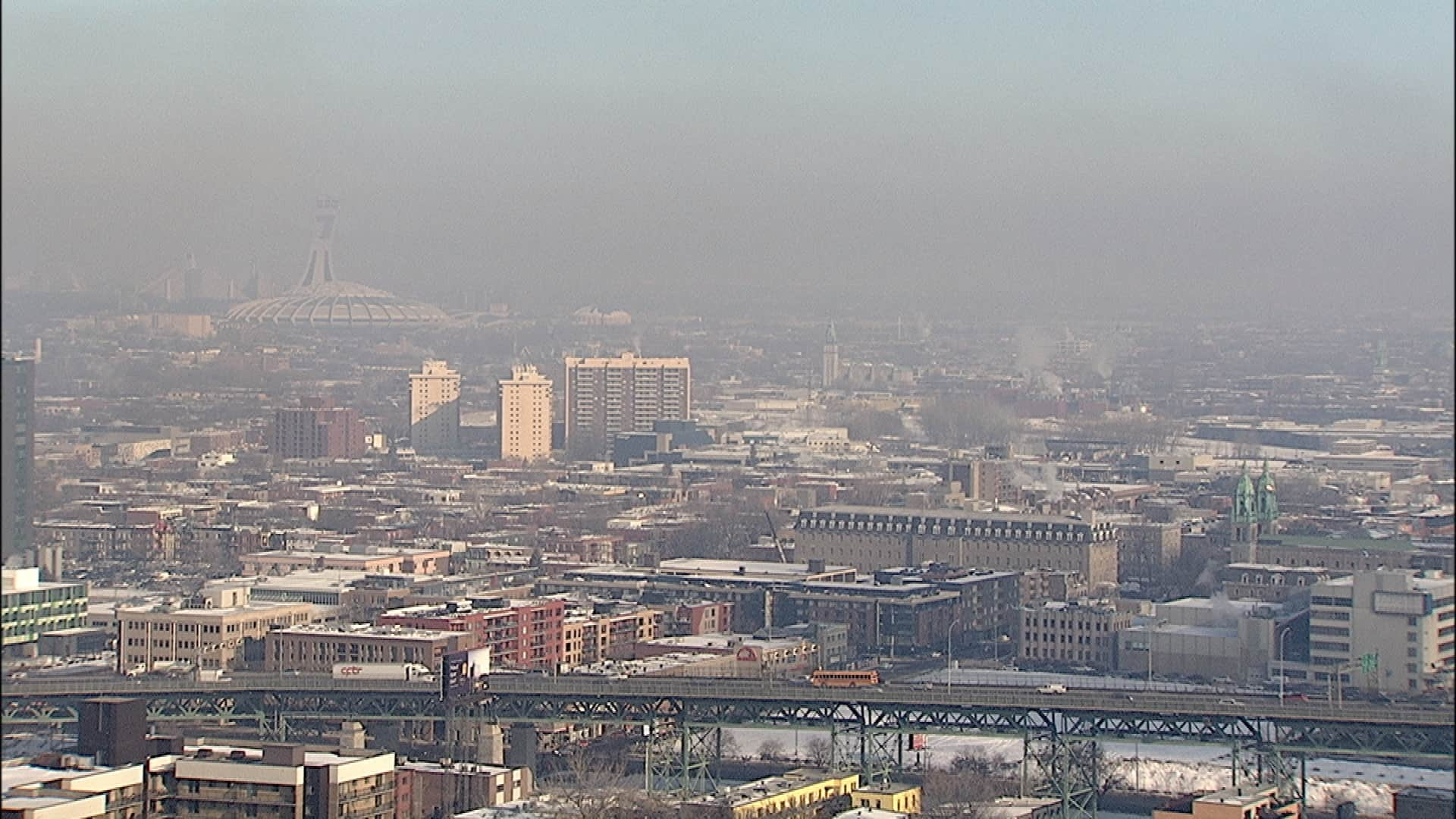This aerial photograph captures a densely packed cityscape shrouded in thick smog, which obscures the background and gives the sky a dark, bluish-gray hue. The city's buildings are primarily tan, brown, and red, interspersed with a few distinctively colored structures like a green building in the lower left and a yellow one in the lower center. The buildings vary in height, with most being multi-story, but not quite skyscrapers, typically around five or six floors. Dominating the foreground is an elevated highway, extending from left to right and curving slightly upward, where several cars, including a noticeable orange school bus, are visible.

A large, segmented dome structure emerges faintly in the smoggy distance, along with sporadic smoke emanating from some buildings, adding to the industrial feel of the scene. There are also a few statues barely discernible through the haze. Overall, the scene looks dirty and heavily industrial, with few trees, and those visible are barren, suggesting a colder season. The smog considerably reduces visibility, making the city's far reaches appear blurry and indistinct.